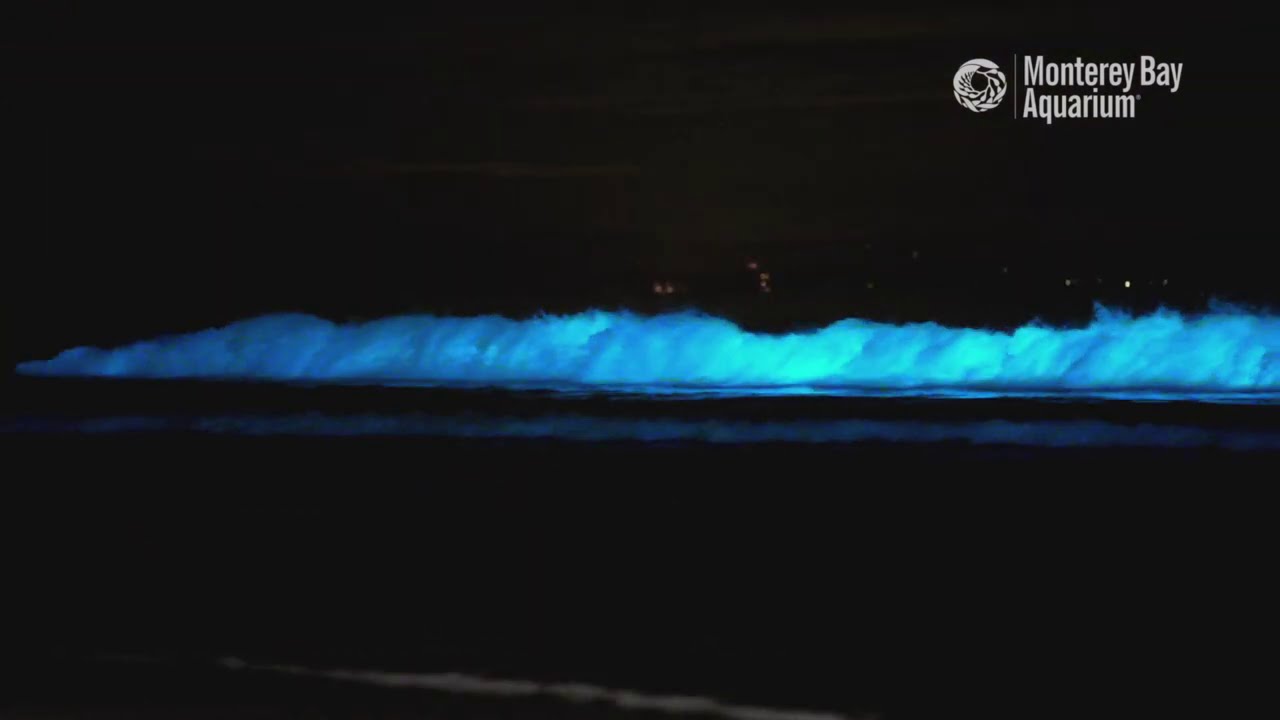This is a nighttime photograph taken at the Monterey Bay Aquarium, as indicated by the white text in the top right corner of the image. The scene is predominantly pitch black, with the most prominent feature being a tall, fluffy white object in the water that looks like a quickly moving wave, its reflection visible on the surface. In the upper part of the photograph, a solitary dark cloud is barely discernible against the night sky. Dim, orange glowing lights are scattered faintly in the distance, while a fairly bright light is more prominent on the right-hand side of the image. Additionally, the silhouette of a mountain range can be made out in the distant background. The photograph appears to have been taken from behind a rail, which is vaguely visible at the bottom of the frame. The overall shape of the image suggests it might be part of a poster, being rectangular rather than square.